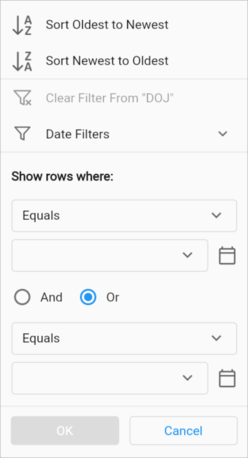This image displays a screenshot of a website interface featuring an options pop-up for managing data filters. At the top of the pop-up, there are two sorting options: "Sort oldest to newest" and "Sort newest to oldest." Below these options, there's a section labeled "Clear filter from DOJ Date Filters."

In the main body of the pop-up, there is a heading, "Show rows where," followed by a dropdown box containing the option "equals." Adjacent to this dropdown, there is a small, empty clear box with a calendar icon next to it, indicating that users can select specific dates. Additionally, there are toggle options labeled "and" and "or," each accompanied by their own dropdown boxes and calendar icons.

At the bottom of the pop-up, there are two buttons: "OK" and "Cancel," facilitating user actions. The interface appears to be designed for managing and sorting data within a spreadsheet or graph application, allowing users to filter data by specific criteria. The color scheme is simple, featuring white, light blue, and gray tones. The calendar icons suggest the functionality to select specific dates for filtering data.